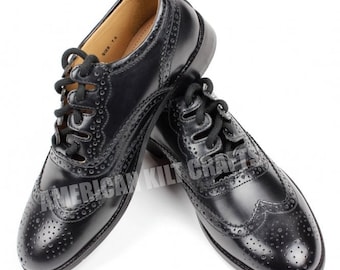The image features a pair of glossy black men's dress shoes, characterized by their wingtip design with decorative broguing. Each shoe is adorned with tiny perforations around the laces and across the toe area in a scalloped pattern. The shoes, made from a shiny, patent-leather-like material, have black laces and stitching. The interior is a contrasting tan or khaki color. One shoe is positioned with its heel resting inside the opening of the other shoe. Overlaid on the image is a light watermark that reads "American Kilt Crafts."